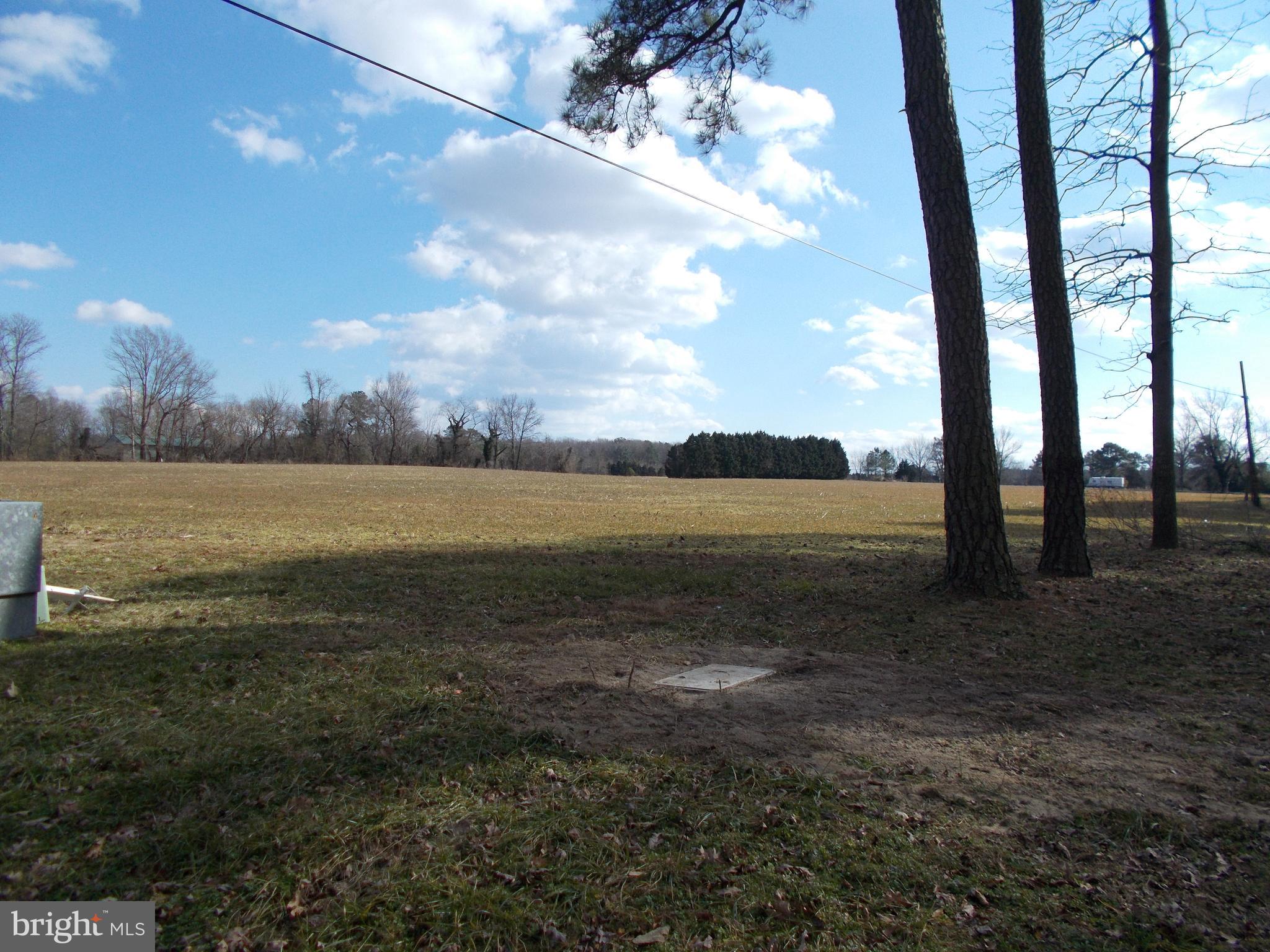This photograph captures an expansive, empty grassy field under a bright, midday blue sky dotted with fluffy white clouds. The field, with its mix of brown, green, and yellow hues typical of fall or late winter, stretches back to a backdrop of numerous trees, most of which are barren, hinting at the changing seasons. Interspersed among these are a few pine trees, and the ground is scattered with fallen leaves. A power line crosses the field, with the pole standing closer to the left side of the image. On the right-hand side, the trunks of three trees stand distinct, with the nearest being the largest and each progressively smaller. The smallest tree exhibits branches lower to the ground. In the center of the field lies a noticeable dirt patch with a white square, possibly resembling a baseball base or plaque, resting on the ground. To the left of the image, a small metallic structure or shed peeks into the frame, adding a hint of intrigue as its purpose remains unclear. The entire scene is bathed in the bright light of day, highlighting the textures and contrasts of this serene, open landscape.